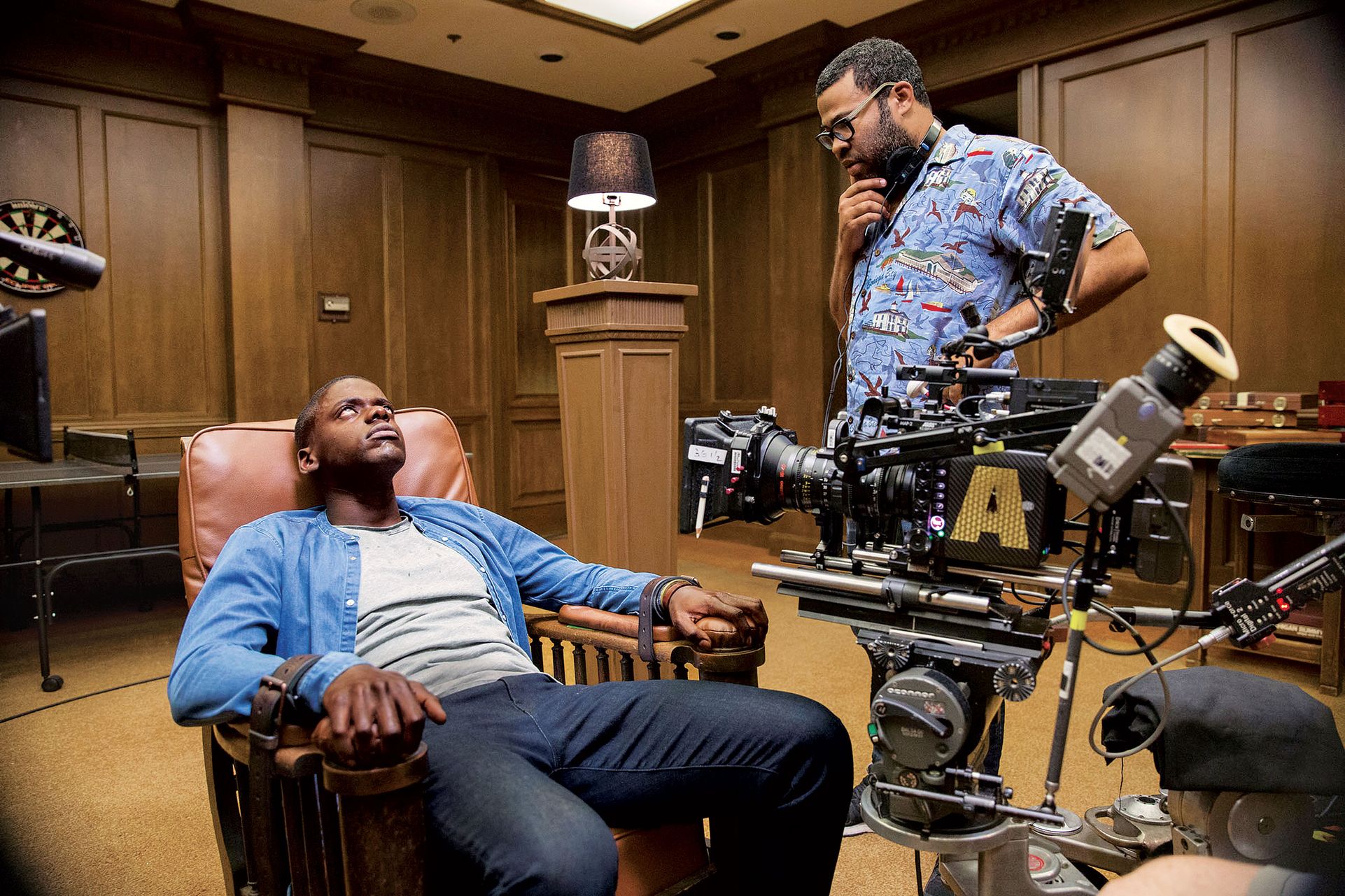This color photograph, taken on the set of Jordan Peele's movie "Get Out," features two African-American men in a detailed scene. One man is sitting in a brown leather chair with his arms strapped to the armrests with leather belts. Wearing a denim jacket, gray shirt, and dark blue jeans, he appears to be in a trance, staring upwards at the ceiling, seemingly detached from the surroundings. He has short-cropped hair and a small amount of facial hair on his chin. Positioned next to him is a complex device, possibly a camera or medical apparatus, marked with a large letter 'A.' 

Standing behind this device is another man, identified as Jordan Peele, the director of the film. Peele, who has short hair and more extensive facial hair that extends to his ears, is wearing glasses and a distinctive blue shirt adorned with images of buildings and various objects. He looks inquisitively down at the seated man, while a headset hangs around his neck. The setting is an all-wooden room with lights on the ceiling and platforms, as well as a dartboard visible in the back left.